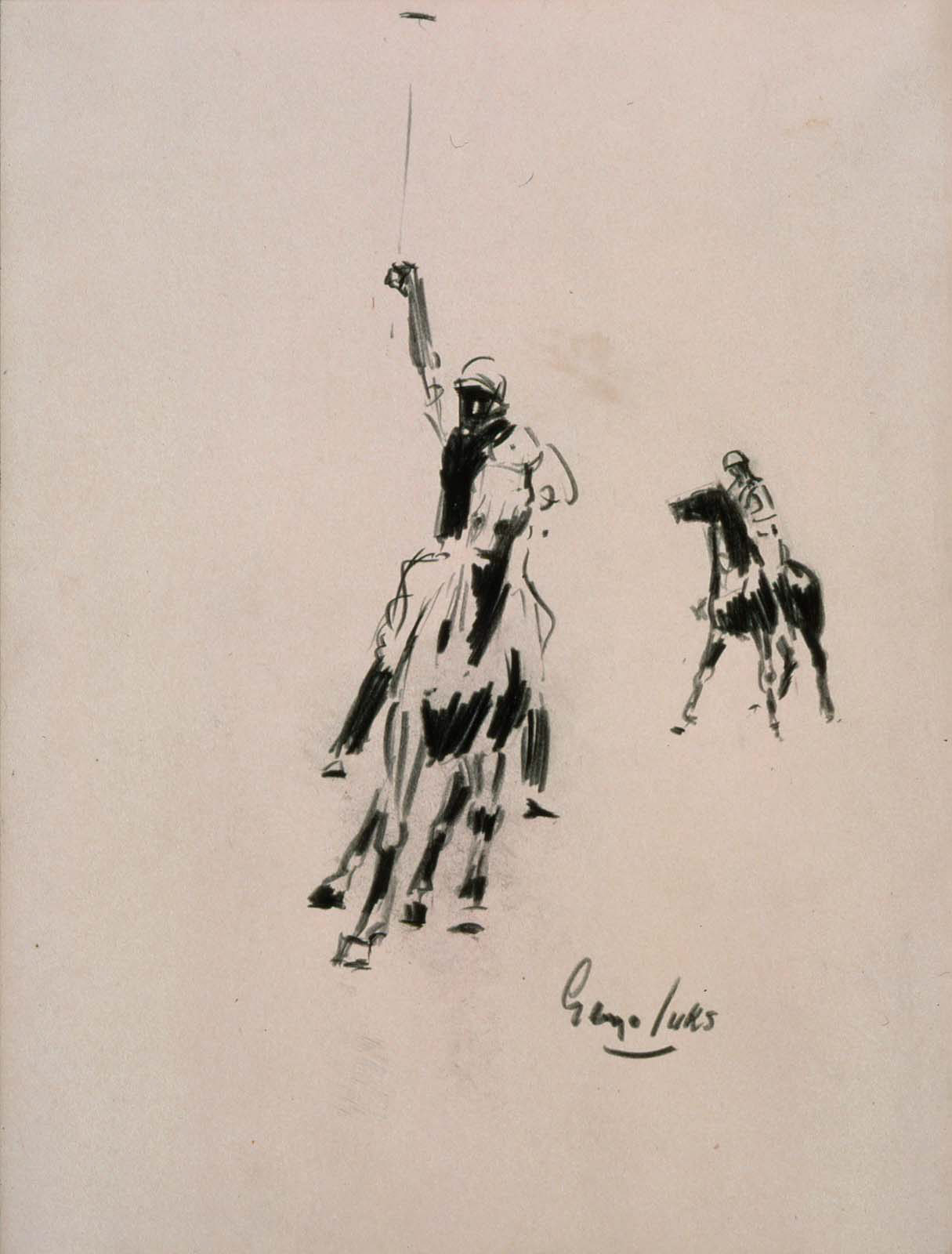The image is an abstract drawing, possibly rendered in marker or pencil, depicting two men playing polo on horseback. The background is a beige color, and the paper appears plain with the drawing in various shades of black. In the foreground, a man is prominently featured riding a horse in motion, wearing a dark riding outfit and a helmet. His arm is raised, holding a long stick, likely a polo mallet. To the right, another rider and horse are sketched, appearing significantly smaller to suggest distance. The scene includes the artist's signature, possibly reading "G-L-Y-O-L-U-K-S," located at the bottom right-hand side of the drawing. The composition emphasizes the dynamic posture of the main player in the middle, while the smaller figure in the background gives depth to the piece.